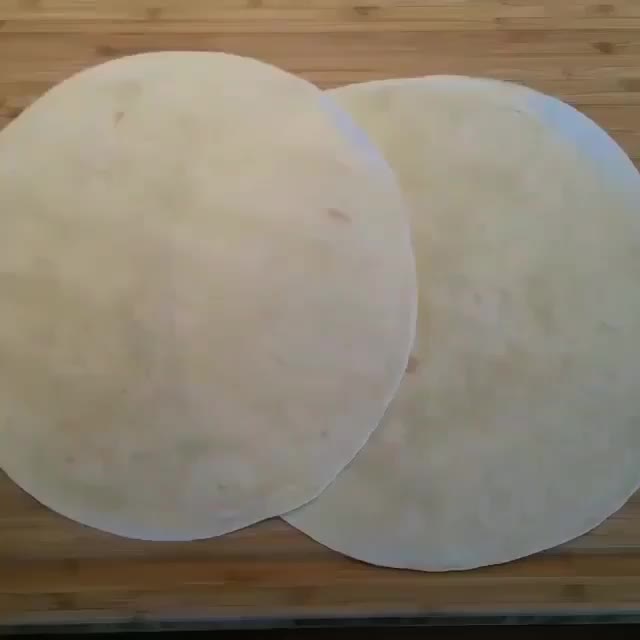This photograph captures a close-up view of a light-colored wooden surface composed of narrow, tightly-fitted planks, devoid of visible gaps. A distinct black line runs along the bottom edge, hinting at a background beneath the wooden surface. Centered in the frame are two large, perfectly round flour tortillas, each approximately six inches in diameter. The tortillas are stark white with tiny brown spots and appear uncooked, as they lack any signs of being on a stove. One tortilla partially overlaps the other on the left side, both seemingly laid out in preparation for filling. The scene is dimly lit, suggesting that the photo may have been taken in the evening, with the overall ambiance casting a subtle shadow over the setting.